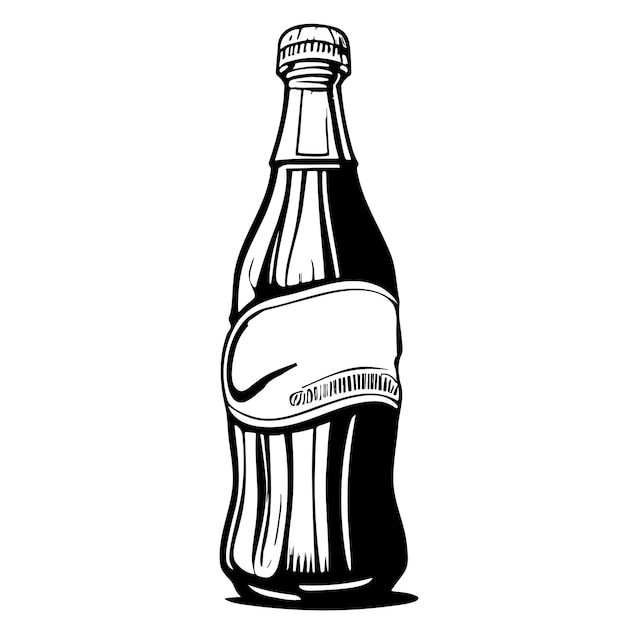This black and white cartoon-style drawing depicts a glass soda bottle with a simplistic, two-dimensional design, similar to ink illustrations. The bottle, standing upright, has a screw-off white cap and a neck that's slender at the top, which widens gradually down to the base. The top of the cap features a black stripe with adjacent downward-pointing black lines. The bottle is mostly filled with an undetermined liquid, as the shading suggests the possibility of a dark substance. A prominent feature is the white label in the center, bordered by a thin black line, which spans from left to right and appears unbranded except for a barcode-like pattern on the left that resembles a dark 'C'. There is shading to the right of the bottle and beneath, indicating light source from the left, and a minimal shadow at the base accentuates its presence. Overall, the bottle's design is reminiscent of a classic glass Coke bottle, emphasizing its curves and unembellished aesthetic.